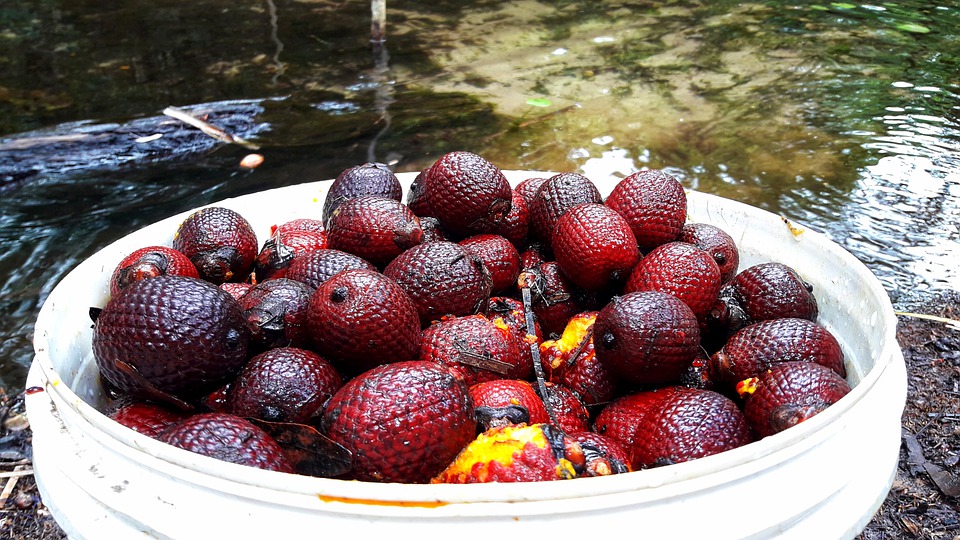This photograph captures a picturesque scene at the water's edge, where a large white bucket, possibly plastic with a screw-on lid, sits on the dirt and debris of a river or lake bank. The water behind the bucket is clear and reflects various natural elements like trees and underwater plants, showcasing ripples and a sandy bottom alongside a large stone protruding into the water.

Inside the bucket, there is a heap of peculiar, dragon egg-like fruits. These fruits vary in shades, from bright red to darker red, and have a scaly, dimpled texture reminiscent of dragon skin or large raspberries. Some fruits are broken open, revealing their bright yellow, peach-like flesh. This unusual fruit, foreign to typical U.S. produce, appears melon-sized and carries an intriguing mix of colors, including splotches of black and yellow on some pieces. The scene suggests an outdoor, possibly cultivation-related activity near the serene body of water.